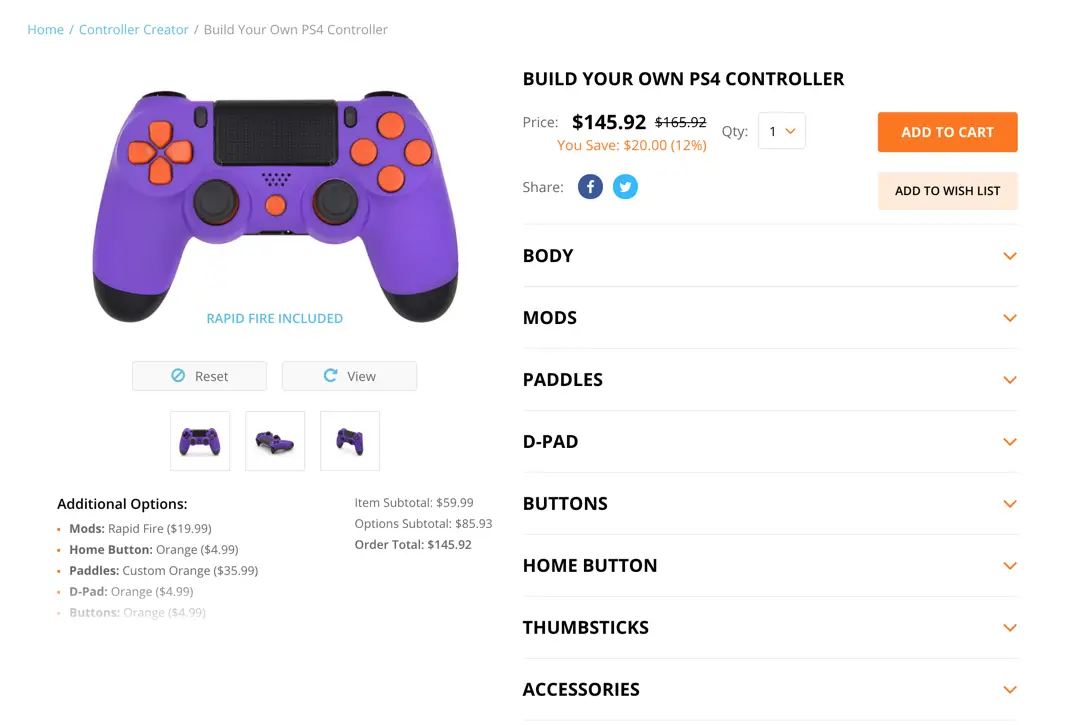Here's a cleaned-up and detailed caption for the image described:

"This image showcases a custom PlayStation 4 DualShock 4 controller available for personalization on a website. The controller prominently features orange face buttons and black analog sticks. The touchpad and triggers, along with the option and screen capture buttons, are black. The top casing of the controller is a vibrant purple, while the back portion is black. The page background is white, providing a clear presentation of the controller's custom features. Beneath the main image, there’s a label indicating 'Rapid Fire Included,' along with reset and view buttons, and several smaller images displaying the controller from different angles. Additional customization options are displayed below the main image. On the right side, the text reads 'Build Your Own PS4 Controller,' with a price of $149.92, indicating a savings of $20 or 12%. 'Add to Cart' and 'Add to Wishlist' buttons are also located on the right. Below these, the sections for customization are listed: Body, Mods, Paddles, D-Pad, Buttons, Home Button, Thumbsticks, and Accessories."